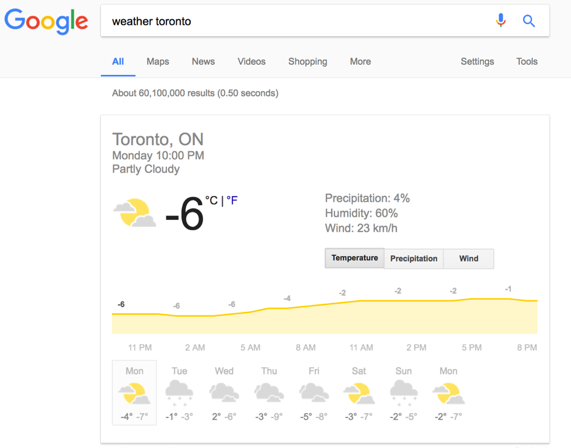A collection of recording devices, possibly old-fashioned tape recorders or modern digital recorders, is scattered on a table, their buttons and dials prominently displayed, capturing the vintage and technological essence of sound recording.